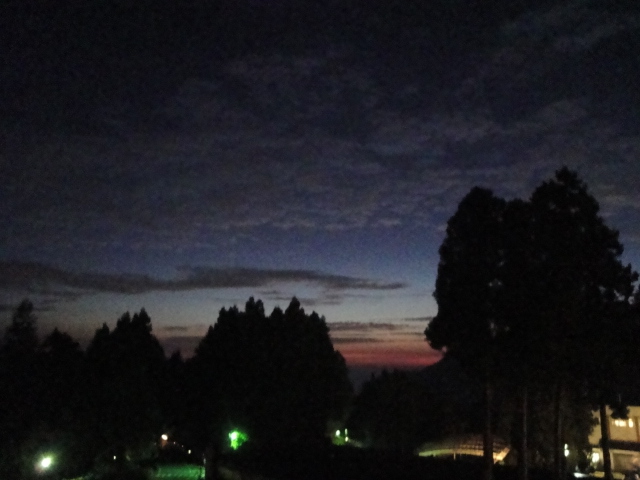The image captures an outdoor scene during late evening, highlighted by a predominantly dark sky with hints of lighter blue and pink near the horizon, suggesting a recent sunset. The upper portion of the photo is occupied by a vast sky filled with numerous clouds, while the lower part features shadowy silhouettes of large trees. In the bottom section, various buildings can be seen, albeit faintly due to the dim lighting. A notable detail includes a string of lights ascending diagonally, likely reaching towards the roof of a building, accompanied by a prominent beam of light. Additional light beams and rectangular sections of illumination suggest the presence of apartment windows or another type of building structure. The scene is brightly colored with hues of black, dark blue, gray, white, green, yellow, and tan, but it remains clear that no text, people, or vehicles are visible. The photograph, taken from a vantage point seemingly high off the ground, offers a clear and high-quality visual of this transitional time of day.